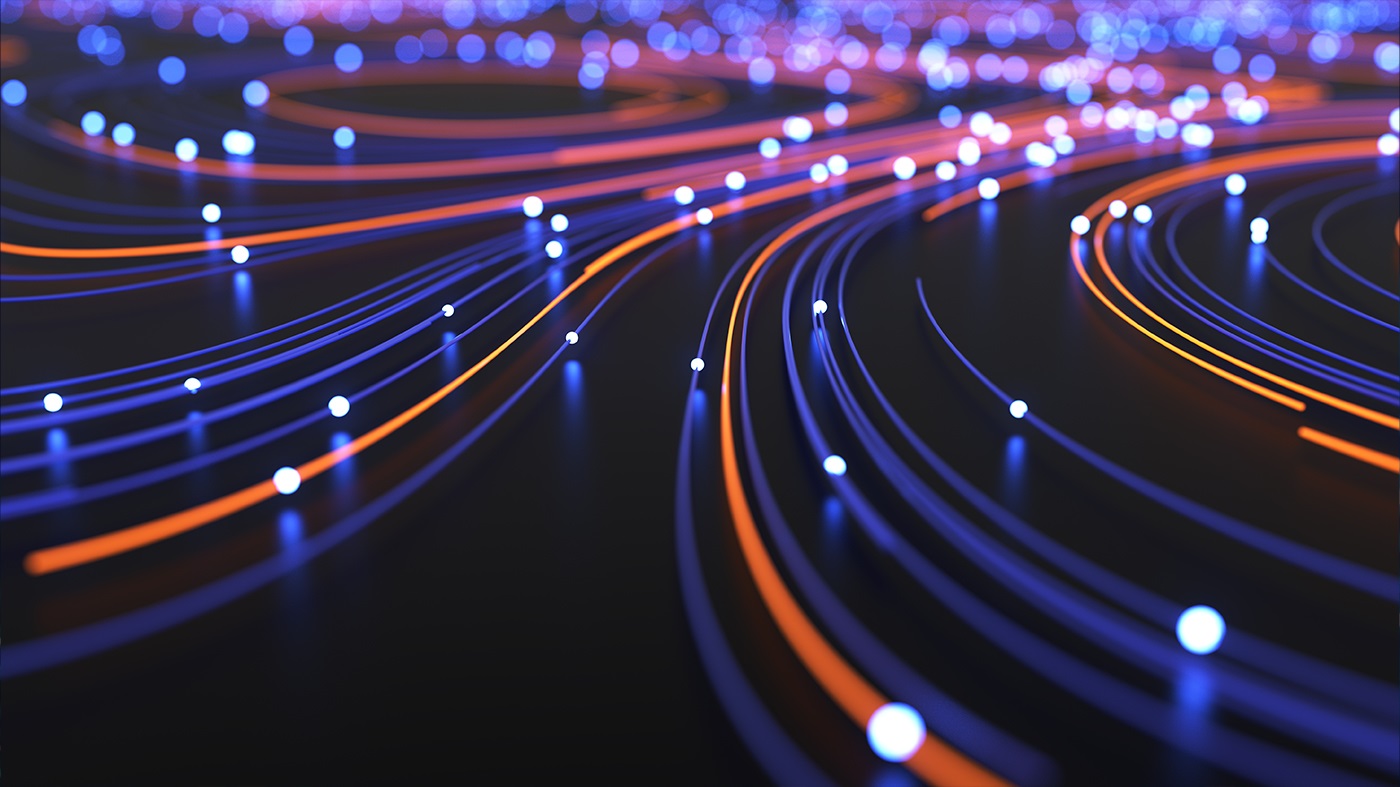This abstract image, potentially a digital graphic design or a long exposure photograph, features a mesmerizing array of fiber optic-like streaks in vibrant colors. The composition showcases a flowy, spiral pattern with streaks predominantly in shades of blue—from light to dark—and various hues of orange, sometimes blending into yellow-orange. These streaks extend from different parts of the image, including the lower right corner and the left center, converging towards a central upper area. Throughout the dark, almost black background, numerous white circular dots punctuate the streaks, creating the impression of tiny, out-of-focus lights. This intricate dance of colors and light gives the image a sense of motion and depth, evoking the complex, concentric design of a pinball machine with its multi-colored lines and luminous details.